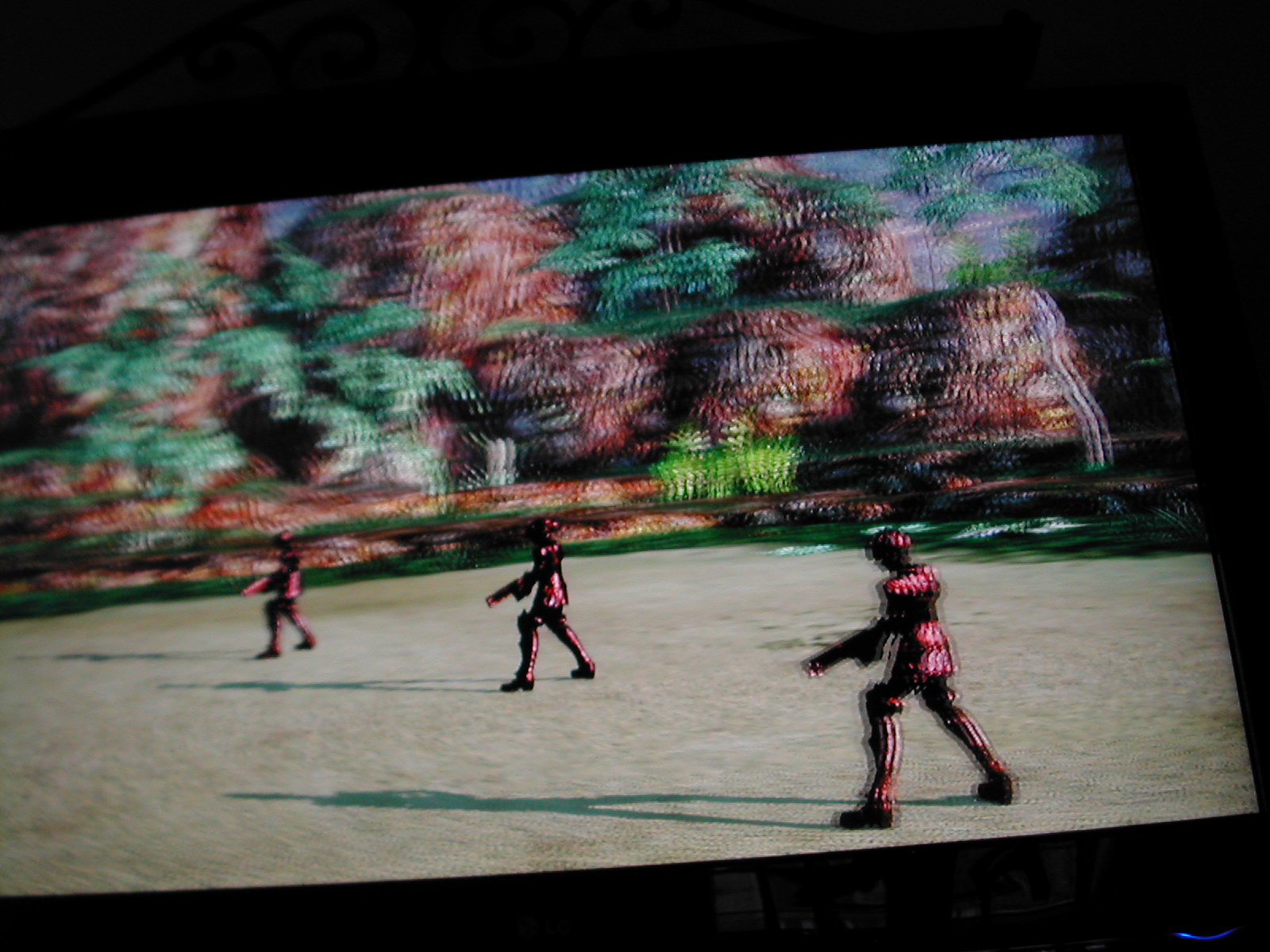The image captures a photograph of a TV or computer screen displaying a video game, resembling the style of older Final Fantasy games and showcasing a combat scene. The foreground features three soldiers dressed in metallic red armor, holding large guns, and casting long shadows to the left. Each soldier stands about five to six inches apart on a sandy surface. The background depicts a highly pixelated, mountainous area with polygonal red-hued mountains, lush green vegetation, and tropical elements like palm trees and possibly cacti. A coastal vibe is suggested by the setting, despite the absence of visible water. Additionally, a blue light at the bottom right corner might be from the game console or TV.